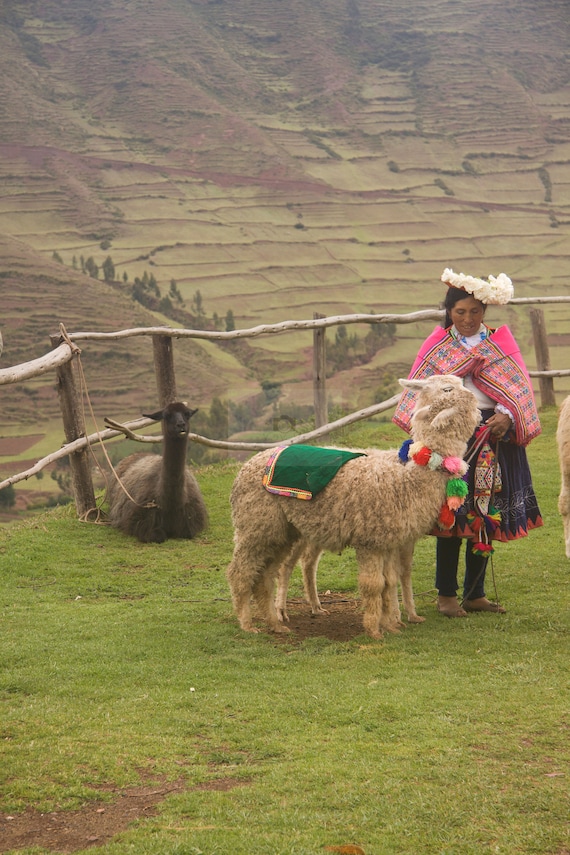In this vibrant photograph taken in the Andes Mountain Region, a woman in traditional Andean attire poses next to two llamas within a grassy enclosure bordered by a rustic wooden fence. The backdrop reveals a picturesque landscape with a mountainside cascading down, covered in patches of greenery interspersed with touches of brown.

At the center of the image, a white llama stands adorned with a green fabric draped over its back and a colorful lei composed of blue, yellow, red, and green ornaments encircling its neck. Beside this llama stands the woman, dressed in a white shirt adorned with a pink shawl that features orange and blue detailing at its edges. She wears a round hat decorated with white flowers, a deep blue skirt with pink trim, and blue jeans tucked into brown shoes.

To the left, a dark brown llama lies flat on the grassy ground, tethered to the fence with a rope. This llama gazes directly at the camera, while the woman appears engaged with the white llama, smiling and looking downward.

In the far distance, the mountainside hints at cultivated farmland, further enriching the scene with a textured, horizontal rippling pattern that completes this stunning depiction of rural Andean life.